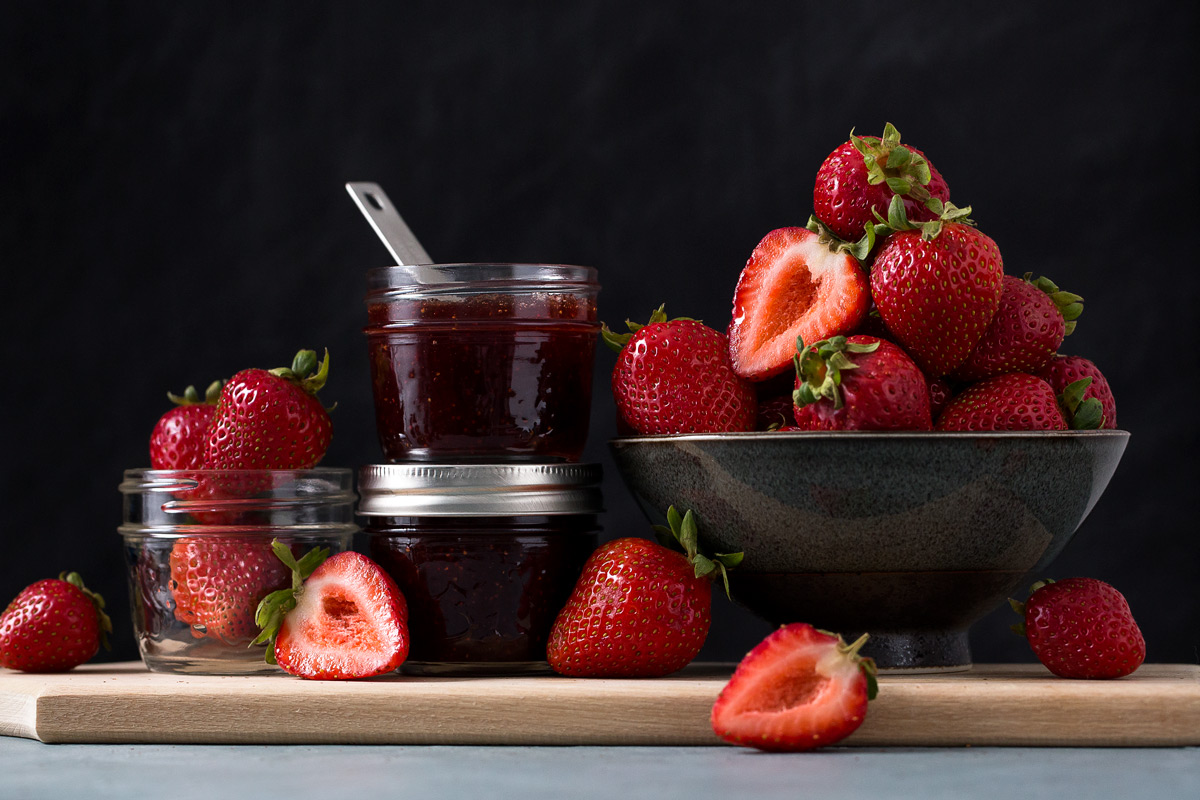The image showcases a meticulously arranged display of strawberries and strawberry jam set against a dark, deep black background. The focal point is a dark-colored, silver bowl filled with an ascending pyramid of strawberries, which is positioned slightly right of center on a wooden cutting board. The pyramid consists of nine strawberries: one at the top, two in the middle, and five at the bottom. Among these, one strawberry is distinctly cut in half, its other half lying in front of the bowl on the wooden surface, surrounded by two whole strawberries — one to the left and one to the right of the bowl.

To the left side of the image, there is a small glass jar with three whole strawberries sealed inside. Adjacent to that, two jars of strawberry jam are stacked, the top jar opened with a small spoon sticking out. Both elements rest on the same wooden cutting board that holds the bowl of strawberries. On the counter, which peeks from the very bottom of the image and appears to be gray concrete, additional strawberries can be seen: one cut in half and another one whole, adding to the visual texture of the composition.